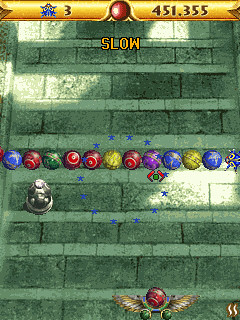A detailed screenshot of a video game is depicted, though the specific game is unknown. At the top of the image, the player's score is prominently displayed on the right side, reading "451,355". In the center of the top panel, a red dot is visible, with a blue star and the number "3" to its left. The word "Slow" is centrally positioned above what appears to be a background of cement or stone bricks.

The bricks are arranged in rows, with each row separated by rows of narrow, rectangular blocks, which widen as they descend. In the middle section of the image, various colored balls with target-like circles on them can be observed; these balls are red, blue, yellow, purple, and green. A symbol beneath one of the balls suggests it might be selected. At the bottom, there is a ball with wings along with something silver beneath the row of colored balls, though the specific details of the silver object are unclear.